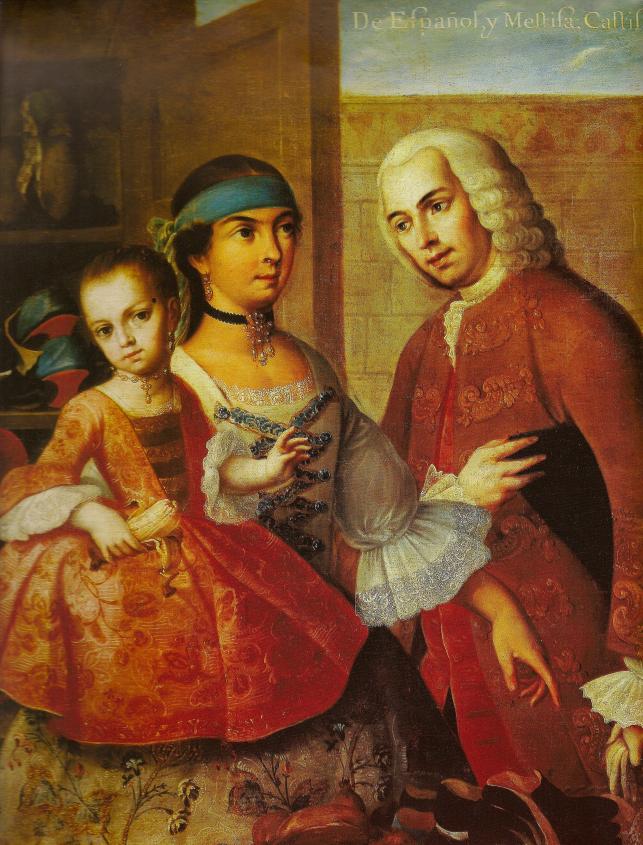This detailed painting, likely from the medieval or Victorian era, depicts an interior scene featuring three characters. On the right side, a man with a powdered white wig that touches his shoulders is dressed in a long, reddish-orange coat adorned with frilly white lace cuffs and a white lace shirt. His right hand, embellished with lace, holds an indistinct object. To his left, a woman stands donning a white and blue dress with green strips of fabric, intricate embroidery, and frills. She wears a blue headband and a choker necklace, with her dark hair pulled back, gazing slightly upward. Beside her, to the far left, a small girl is dressed in a red or orange frilly dress embroidered with floral patterns. Her possible red hair is styled, and she holds what seems to be a yellow piece of paper. The figures’ skin tones are rendered in varying shades of yellow. Behind them, a wooden cabinet filled with various colored objects sits against a reddish stone wall. The top right corner of the painting is marked faintly with the artist's signature, which appears to read "D. Edunoli Malifa Kenif." The background also includes sections reminiscent of skies painted in light blue hues and a wall made of reddish stone bricks, adding to the historical ambiance.